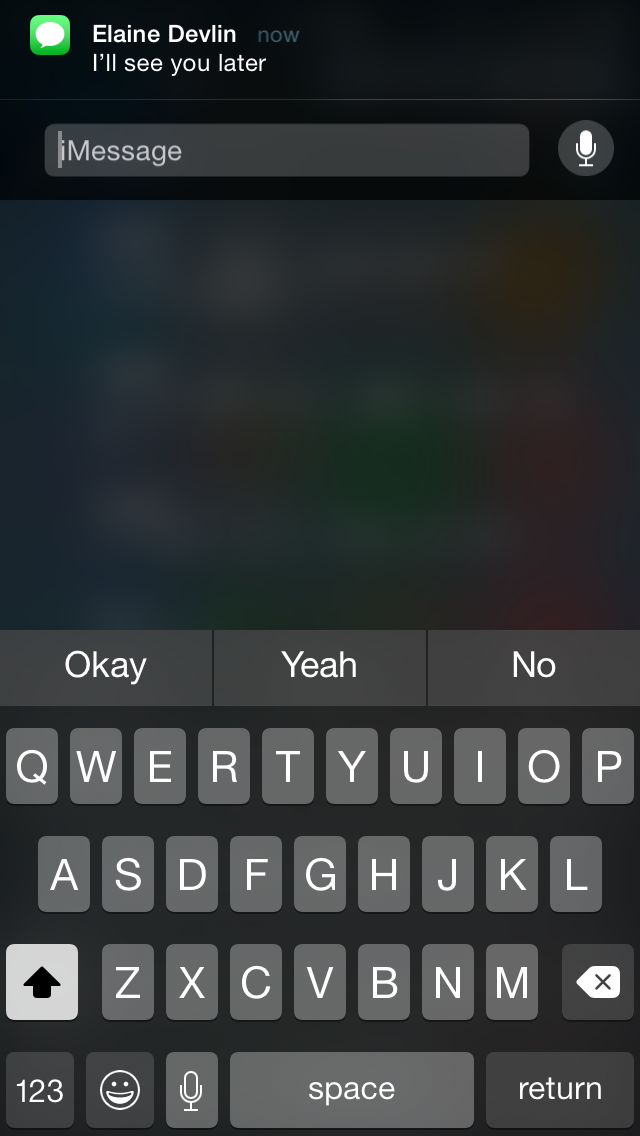In the screenshot, an iPhone screen is displayed, showing a messaging app interface in black and white. A message is being composed with the text input field containing "I'll see you later. Elaine Devlin." Below the text field, there are predictive text prompts that offer quick response options: "Okay," "Yeah," and "No." The keyboard is visible at the bottom of the screen, featuring a full set of alphabet keys, a shift key, and toggles for numbers and emojis, providing a comprehensive typing interface.